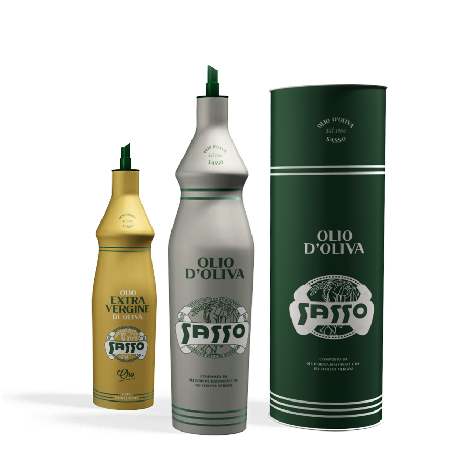This image depicts a product photo of three different olive oil containers from the brand Sasso. The containers are lined up next to each other and each one prominently features the label "Olio D'Oliva Sasso." The container on the left is the smallest, colored gold with the words "Extra Virgin" on the label, though additional details on the label are too small to read. The middle container is the tallest, with a silver design and a porous spout on top, resembling a rocket ship, and carries the same "Olio D'Oliva Sasso" label with illegible smaller writing below. The rightmost container is a deep green canister, also labeled "Olio D'Oliva" and is cylindrical in shape, appearing to be made of paper or plastic. All three containers feature the Sasso logo, which is a banner atop a map, and they have green accents and nozzles.